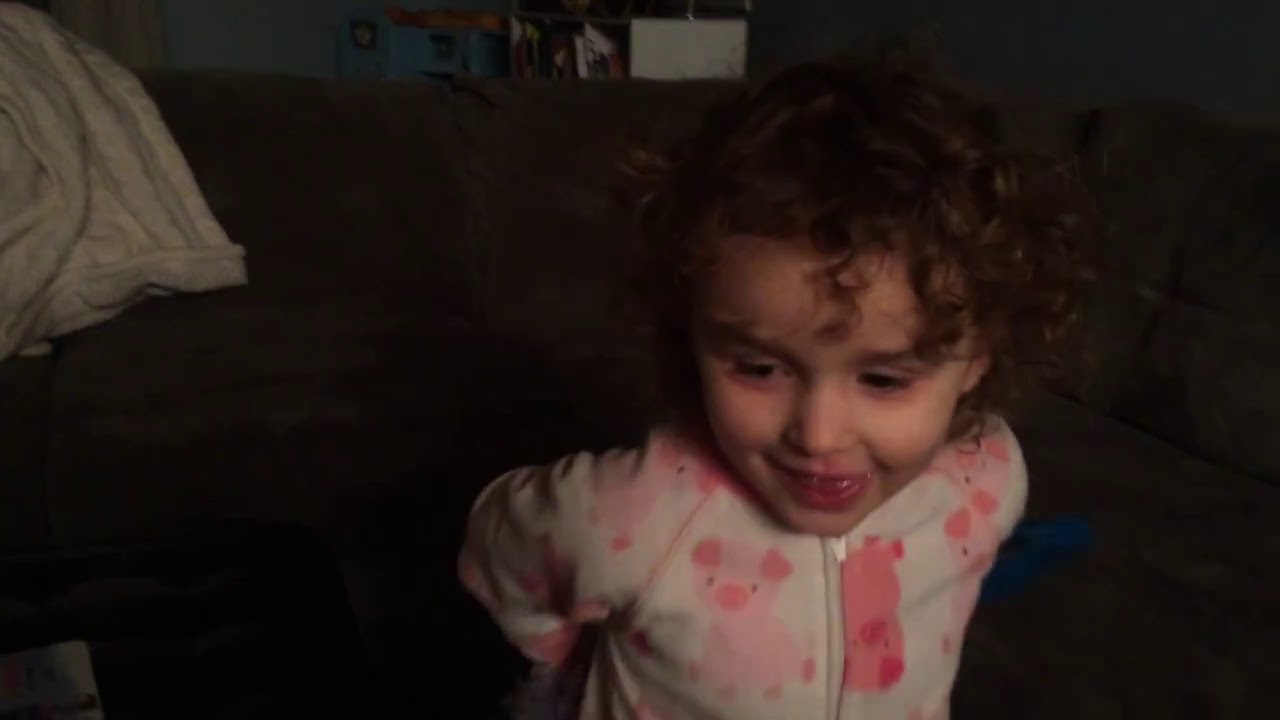In this image, a young girl with extremely curly, reddish-brown hair reminiscent of Shirley Temple stands in the foreground, dressed in a white zip-up onesie adorned with a pattern of cute, pink-dotted pigs. She has a small grin on her face with her tongue playfully sticking out between her lips. The girl appears to be observing something on the floor, slightly to her right. Behind her, the scene transitions to a living room setting with a large, velour-like gray couch that extends in an L-shape to the right of the image. Draped over the left side of the couch is a white and gray blanket. Further back, a beige throw coverlet is flopped over the edge of what appears to be a bed or couch, and beyond that, a bluish wall with shelves holding various items, and a bureau housing a few little statues and a PC monitor adds depth to the background. The ambiance suggests a cozy moment, potentially on a special morning like Christmas, given the girl's excited and cheerful expression.